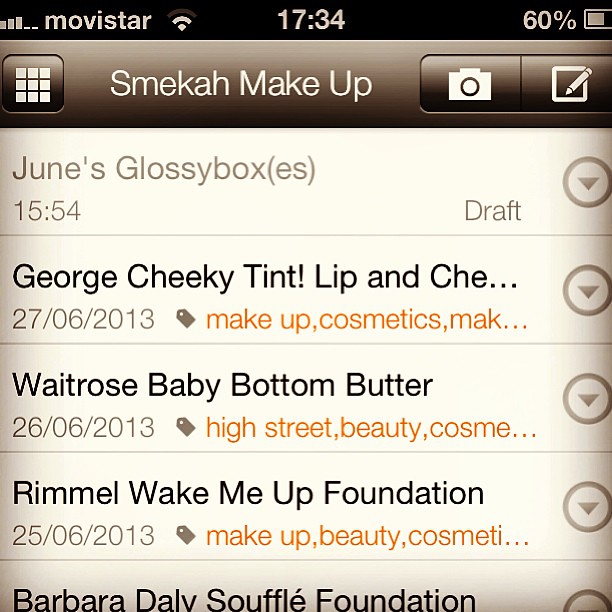The image is a 5x5 inch screenshot from a smartphone app, showcasing a detailed list under a dark brown header. At the top, the blackish-dark brown bar displays "Movistar" with two Wi-Fi bars, the time "17:34", a 60% battery icon, and three signal bars. Below this bar, a medium brown section features "SMEKH makeup" in white text, accompanied by a 3x3 grid icon, a camera icon, and an edit icon.

The main section lists five rows of items related to makeup and cosmetics:
1. **June's Glossy Boxes** (1554) - labeled as a draft.
2. **George Cheeky Tint Lip and Cheek** - with an ellipsis, dated 27/06/2013, and tagged in red with "makeup, cosmetics".
3. **Waitrose Baby Bottom Butter** - dated 26/06/2013, and tagged with "High Street Beauty".
4. **Rimmel Wake Me Up Foundation** - dated 25/06/2013, and tagged with "makeup, beauty, and cosmetics".
5. **Barbara Daly Soufflé Foundation**.

Each item is accompanied by a downward arrow icon, indicating more details or options are available for each entry. The overall appearance is organized and color-coordinated with browns and a touch of orange and red for emphasis. The screenshot comprehensively catalogs various makeup products within a structured digital format.